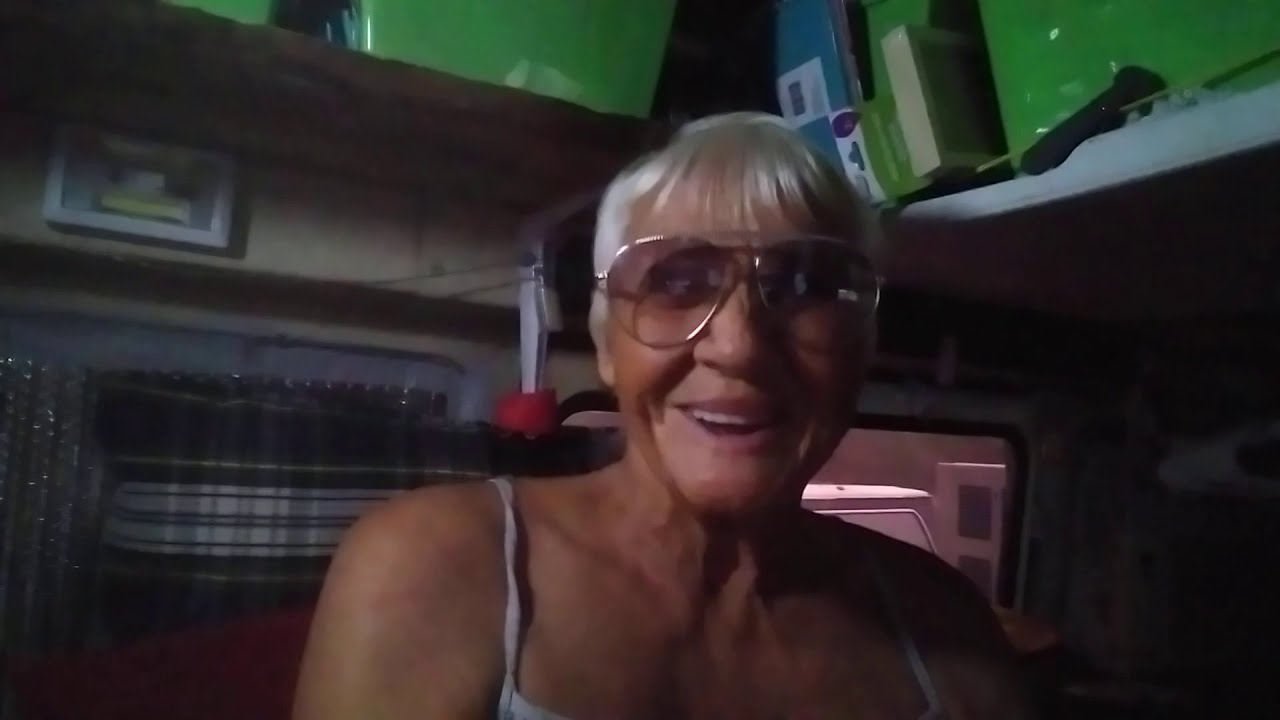The image depicts an older woman, possibly in her late 50s or 60s, inside a dark, enclosed space that resembles the interior of a camper or van. She has short white hair and is wearing large, round sunglasses with pinkish hues. Her complexion is tan, and she is dressed in a white tank top with thin spaghetti straps. The picture captures her smiling broadly, with parted lips revealing her upper teeth, and she gazes slightly to the right. The background shows a small window with a piece of cloth and several shelves at head level, holding green containers. The image is somewhat blurry and out of focus, with a brown and white shelf also visible above her head.